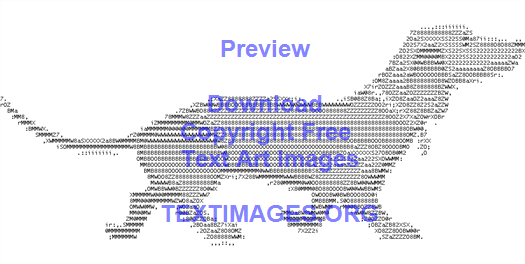The image is a detailed, black-and-white, computer-generated ASCII art depiction of a dachshund (also known as a "doxy" or "hot dog dog") facing right. The dog is illustrated using text characters, showcasing long ears, a slender body, and a long, skinny tail. It wears a collar with a name tag, adding a realistic touch to the artwork. Overlaying the image in purple or blue lettering are the words: "Preview," "Download Copyright-Free Text Art Images," and the website "textimages.org," all set against a white background. The overall style is reminiscent of 80s or 90s retro printouts, blending nostalgia with digital art.